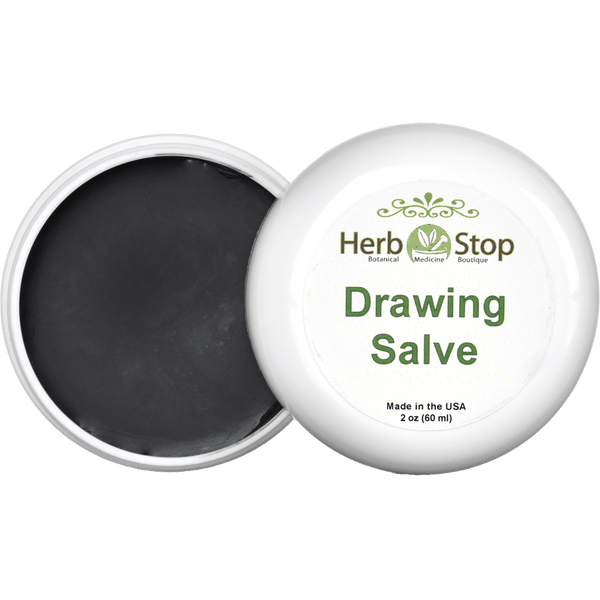The image features a stock photo of a white, round, plastic container of drawing salve from Herbstop Botanical Medicine Boutique. The container's lid is off to the side, revealing a black, matte salve inside. The label on the lid, which is white with green lettering, reads "Drawing Salve" and includes an image of a mortar and pestle with leaves above it, followed by the text "Herbstop Botanical Medicine Boutique." At the very bottom of the label, it states "Made in the USA, 2 ounces (60 milliliters)." The entire scene is set against an all-white background. The salve itself has a slight reflective quality and appears flat. This product seems to be a natural remedy, possibly showcased on the Herbstop website.